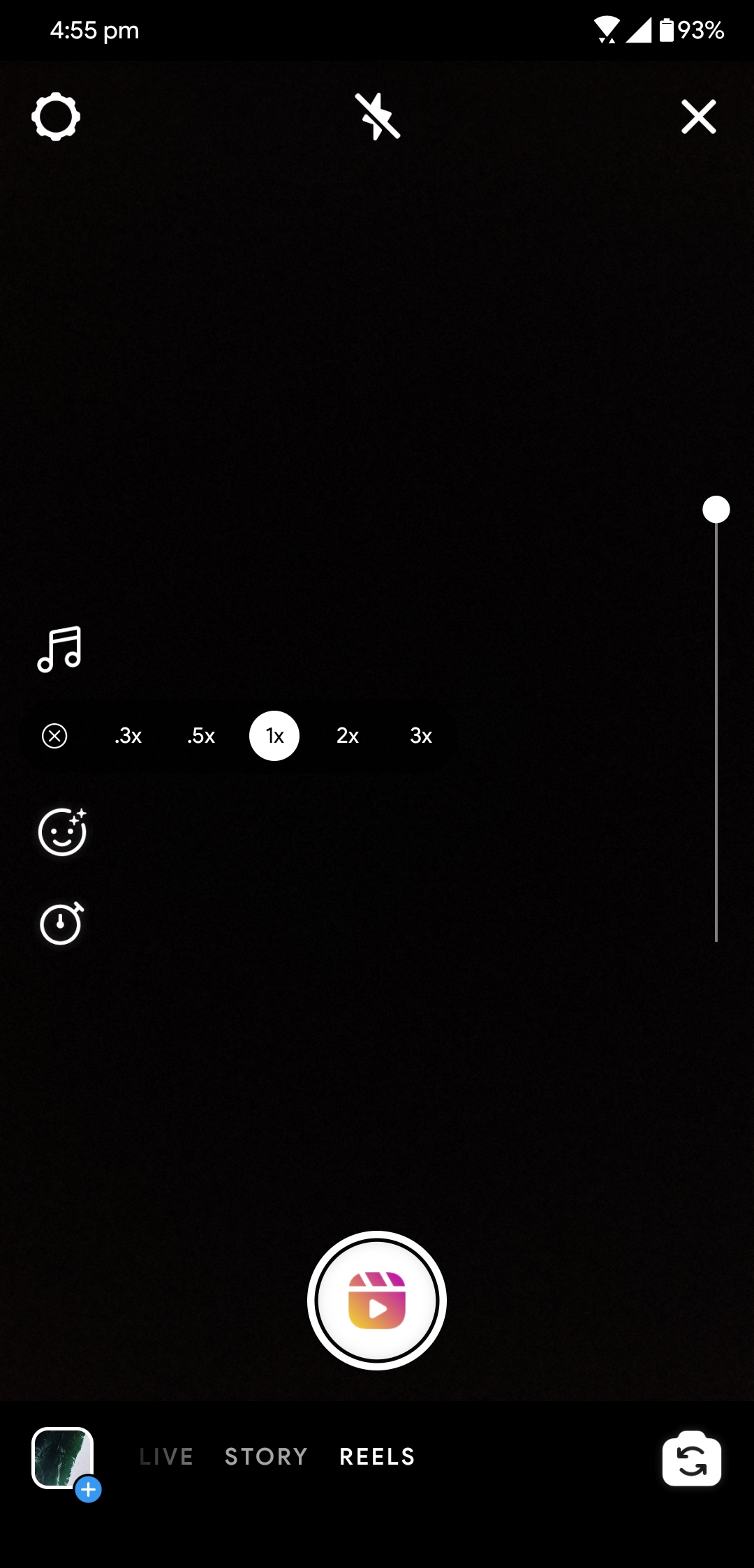A detailed caption for the image:

"This color screenshot was taken from a smartphone at 4:55 p.m. and showcases elements of the device's screen. The top right corner displays a battery life at 93%, with full reception bars. The screen itself reveals the user within their video app, specifically in the 'Reels' section of the camera reel interface. Options at the bottom allow the user to switch between 'Live,' 'Story,' and 'Reels,' with 'Reels' currently selected. The main view of the screen is predominantly blank, appearing black, possibly indicating a loading video or an unpopulated screen. Magnification or speed options are visible, allowing for 0.3x, 0.5x, 1x, 2x, and 3x adjustments, suggesting this is a video editing tool."